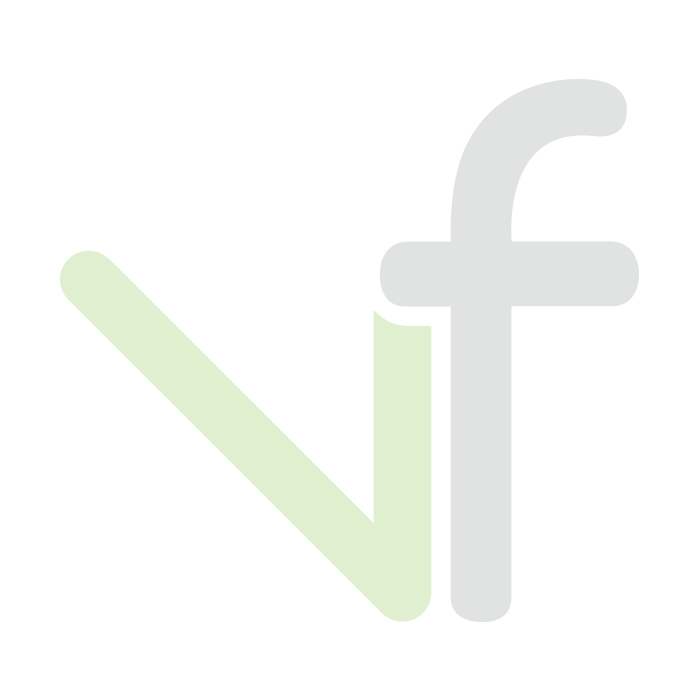This product photo features a colorful and vibrant display of Cloud Nerds Iced flavored e-liquid for vaping. In the image, a 100ml bottle and its accompanying package are shown side by side against a stark white background, devoid of any shadows. The design prominently features a lively mix of bright green, teal, and red colors with abstract shapes that catch the eye. 

Both the bottle and the box share the same logo and design elements, including matching color schemes and fonts. The packaging draws attention with "Cloud Nerds Iced" prominently displayed in white lettering trimmed in blue. Below the brand name, the flavor "Sour Watermelon Strawberry" is split with "Sour Watermelon" in green letters and "Strawberry" in red letters. Important product details are listed, noting that the e-liquid contains 3mg of nicotine and comes in a 100ml bottle. 

The packaging also includes a white warning label with black text stating, "This product contains tobacco-free nicotine. Nicotine is an addictive chemical." The bottle mirrors the box's design and information almost exactly, featuring a clear liquid inside and a practical white cap designed for easy application into a vape pen.